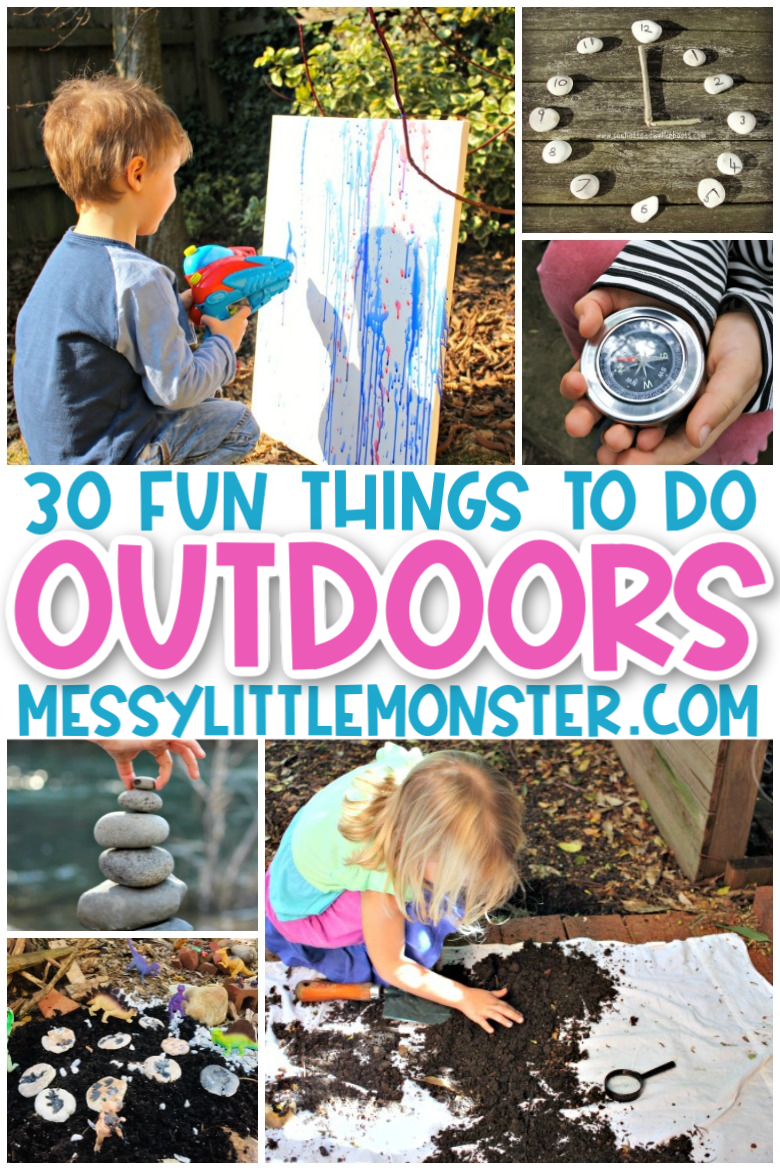This vibrant vertical image, which could serve as a social media graphic, poster, or book cover, features a detailed guide titled "30 Fun Things to Do Outdoors," brought to you by Messylittlemonster.com. The text is prominently displayed in the center with alternating colors of blue and pink. The layout consists of seven photos displayed in clusters on the top and bottom sections.

At the top left, a boy, approximately six years old, is creatively using a squirt gun filled with paint to make art on a white canvas, with vibrant splashes of blue and pink visible. To the right, there's a smaller image of a handmade clock crafted from sticks and stones, alongside another photo of a young child holding a compass.

In the bottom section, on the left side, there are two small pictures: one depicting someone stacking rocks in a garden, and the other showing a garden scene, complete with colorful painted rocks among dinosaur toys. Lastly, the bottom right features a small girl, around six or seven years old, with blonde hair, engaging with black soil and playing with dirt on a white sheet outdoors. This detailed flyer highlights various creative and engaging outdoor activities perfect for children.